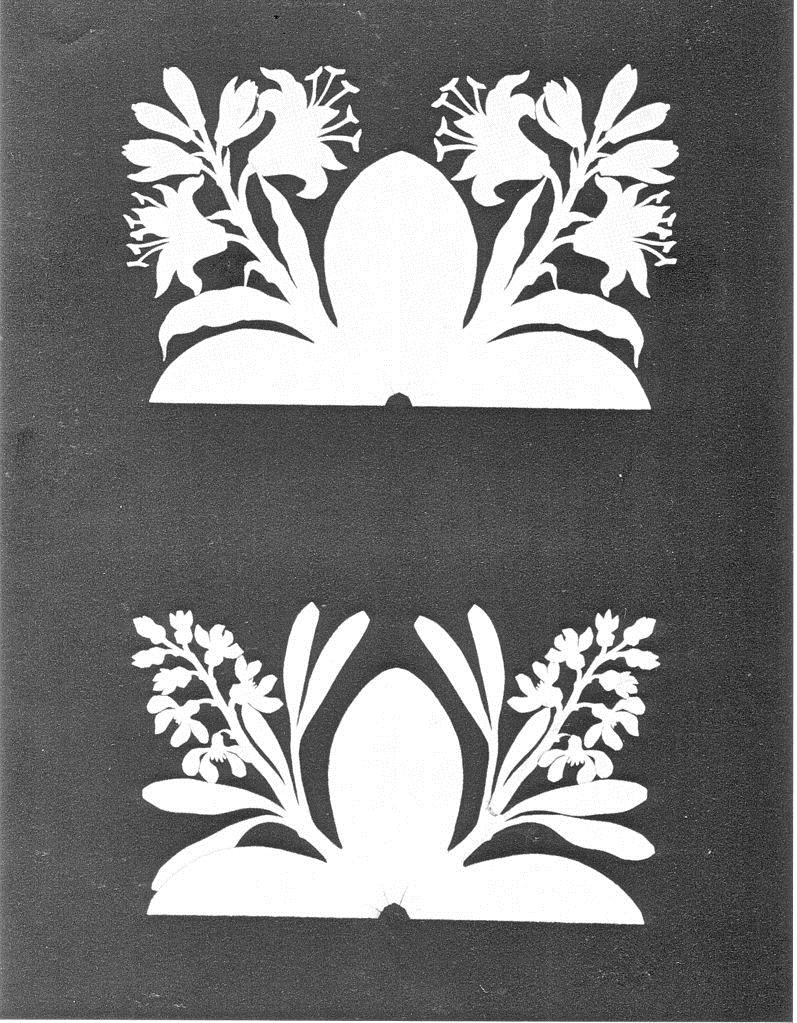This image showcases two intricate white paper cutouts set against a stark black background. Each cutout features a symmetrical design evocative of floral motifs. The top cutout resembles an egg-shaped structure adorned with six flowers—three on each side—where the flowers exhibit prominent petals and stamens. The bottom cutout, also egg-shaped, displays a similar design but features only two larger central flowers with more delicate petals and stamens. Both cutouts appear meticulously crafted, with the flowers branching from a base of three leaves. The backdrop of the image enhances the white cutouts with its sharp, speckled gray texture, giving the artwork an elegant and striking visual contrast.